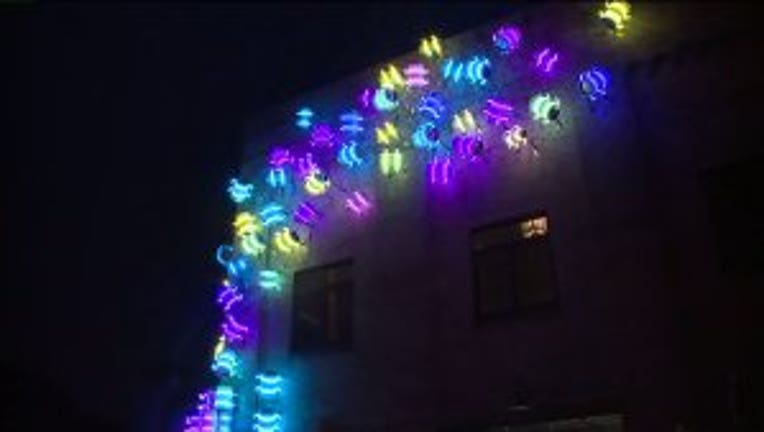In this nighttime image, a white building—possibly an apartment or a factory—stands adorned with a series of large, vibrant lights in shades of purple, yellow, light blue, and blue, forming a diagonal pattern from the bottom left to the top right corner. These lights, approximately basketball-sized, appear to be wrapped with bright LED ropes, creating a striking visual effect against the dark, grainy backdrop of the night sky. The building features two darkened windows, one on the left side and one on the right, adding to the sense of mystery. The overall image quality is low and slightly blurry, but the elaborate light decorations clearly stand out, illuminating the structure in a festive display.